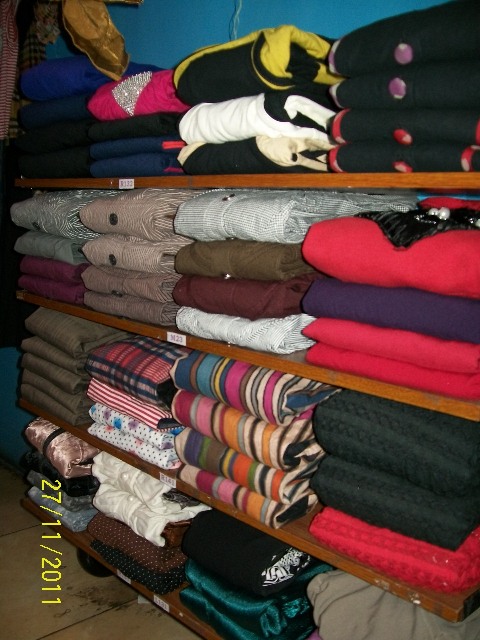This color photograph, marked with a yellow watermark displaying the date "27/11/2011," features a well-organized closet or storage unit against a bright blue or turquoise wall. The vertical rectangular image showcases a wooden shelving unit comprising four shelves, each stacked neatly with a variety of clothing items. The first shelf from the top includes what appears to be dark-colored, possibly black jerseys, and bedding or a sleeping bag in the middle section. The second shelf is filled with different types of clothing, including cardigan sweaters organized in pairs by color and button-front shirts, with a mix of solid and patterned designs. The third shelf presents items resembling brown garments on one side and multicolored striped fabrics, possibly scarves, on the other, alongside green and hot pink clothing pieces. The bottom shelf holds more neatly folded tops, potentially both sweaters and shirts, in various colors. The bright blue wall and the wooden floor, with a noticeable brown stain at the bottom, create a vibrant background for this meticulously arranged display of textiles.